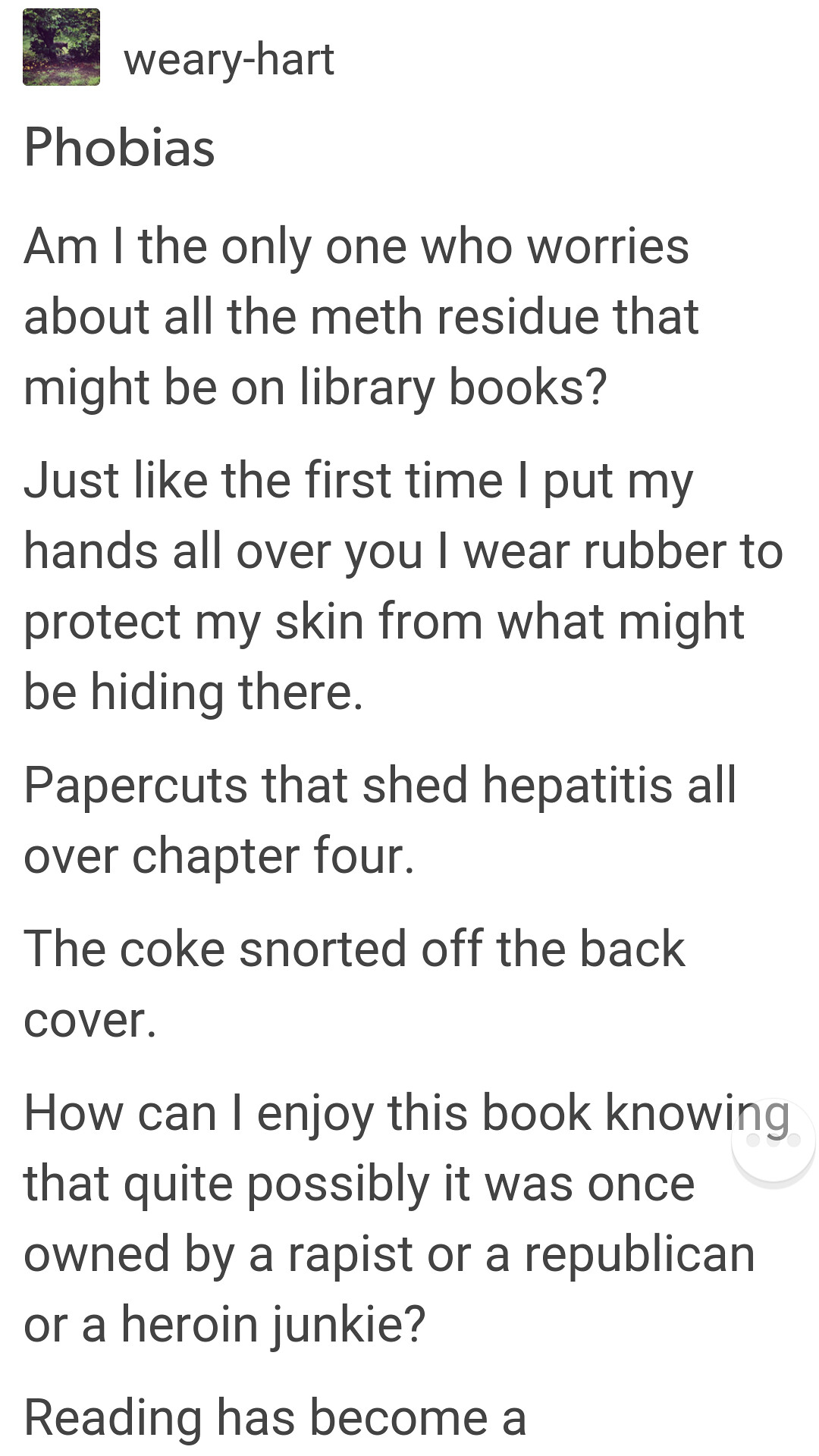This image is a screenshot of a post made on a social media account by a user named Weary Hat. The post, titled "Phobias," is comprised of three paragraphs written in black font on a white background, formatted in sentence case with capitalized beginnings. It reads: "Am I the only one who worries about all the meth residue that might be on library books? Just like the first time I put my hands all over you, I wear rubber to protect my skin from what might be hiding there. Paper cuts that shed hepatitis all over chapter four. The coke snorted off the back cover. How can I enjoy this book, knowing that quite possibly it was once owned by a rapist or a Republican or a heroin junkie? Reading has become A..." The post features a small thumbnail picture in the top left corner, seemingly of an outdoor garden, next to the username and profile icon. The post abruptly ends, suggesting it might be an incomplete entry.